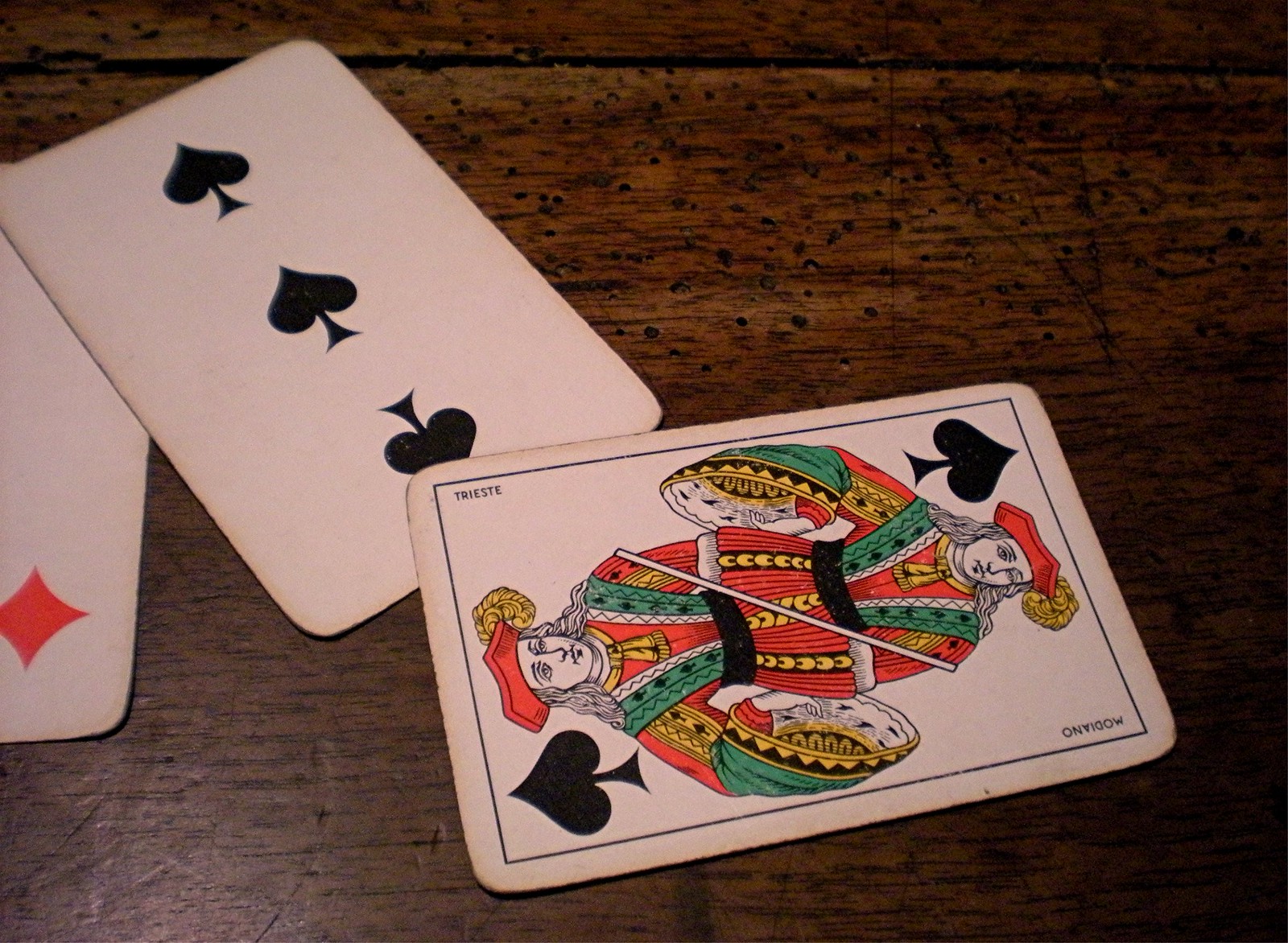A detailed close-up photograph showcases three playing cards arranged on a dark, weathered wooden table. The table's surface, marked by pitted portions and tiny holes, tells of years of use. The cards, with their faded and dingy edges, appear to be vintage and well-handled. 

On the left side of the frame is a card displaying a single red diamond in the corner. Overlapping this is a card with three spades aligned vertically down the middle. Most prominently positioned, yet slightly diagonal from the bottom left to the top right, is a Jack of Spades. The Jack card features a mirrored image of a regal figure adorned in striking colors. The person is depicted in a black and white illustration, set against a vibrant outfit. The Jack wears a red hat with a yellow feather, a red robe with gold collar and accents, and green embellishments down the sleeves. A black belt completes the ensemble. The edges of all three cards reveal signs of age and wear, enhancing the nostalgic feel of the scene.